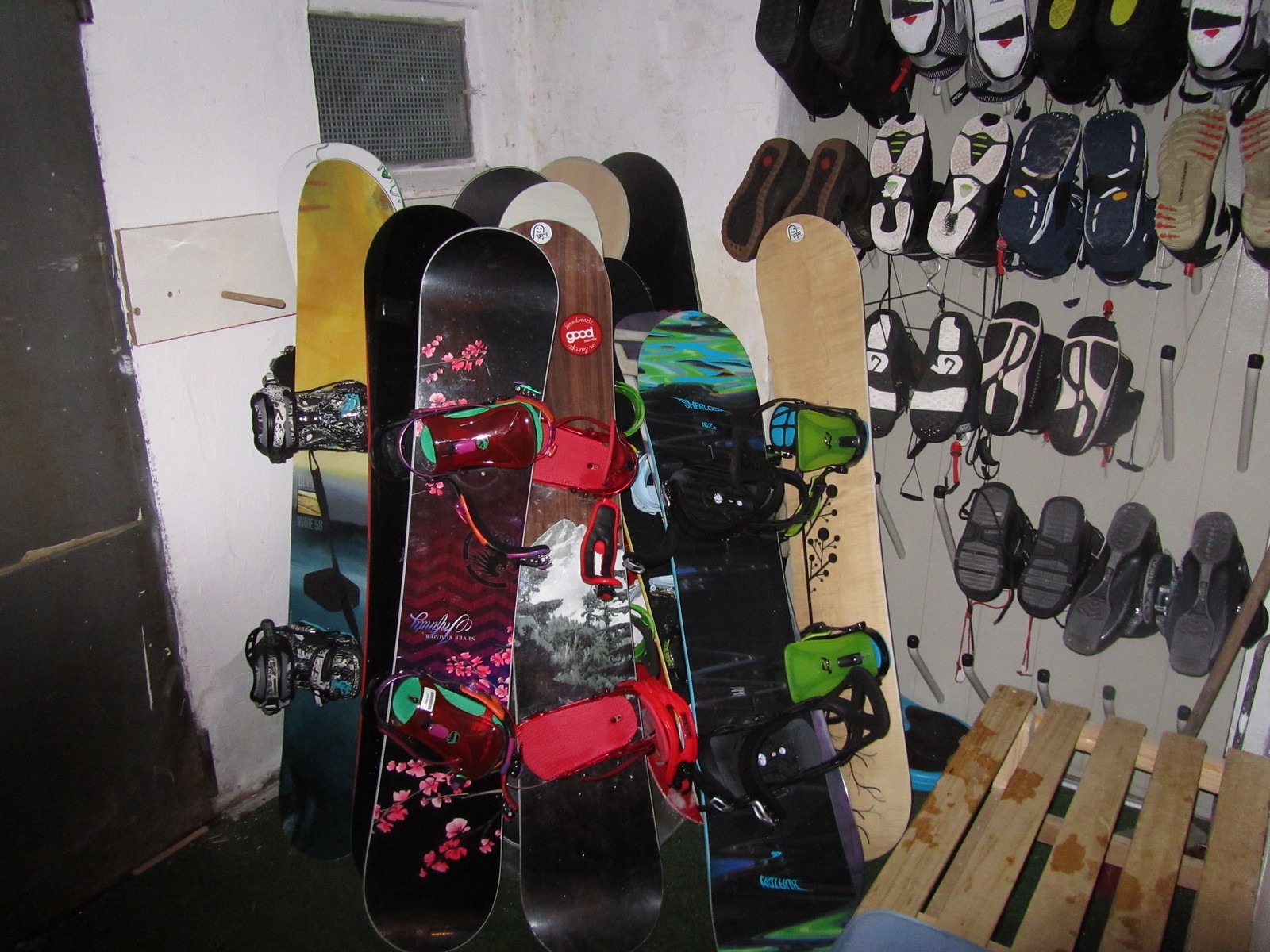The photograph depicts a bustling mudroom, likely part of a business or a ski resort given the abundance of equipment. On the left side of the room, a brown door contrasts with predominantly white walls. There is a gray mesh square above the shoe rack. The focal point of the image is an assortment of snowboards, about eight to ten, propped up against the corner. These snowboards range in color from simple blonde wood to vibrant hues like red, blue, black, yellow, and pink, some with printed designs. To the right of the snowboards, a wall-mounted board features numerous hooks holding a variety of leisure and athletic shoes in colors like black, white, blue, and red. Below the shoes is a simple wooden crate with slats. Additionally, a basic wooden bench is placed in front of the hooks, providing a spot for visitors to set down their belongings. The image captures a well-used space ready for activity.